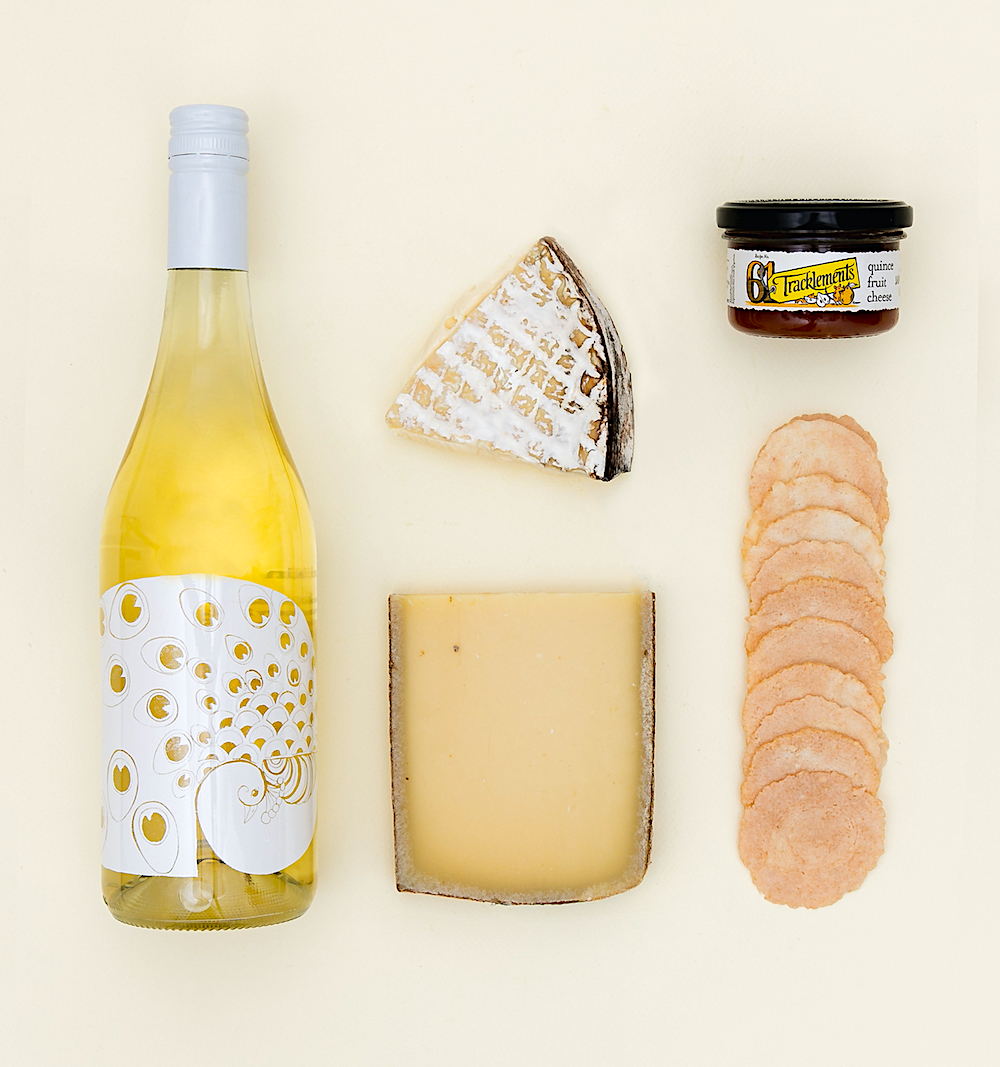The photograph displays an artfully arranged charcuterie board set on a tan-colored surface against a white background. Central to the composition is a large bottle of white wine with an intriguing emblem that resembles a blend of an elephant and a peacock. To the left of the bottle, there's a slice of pie or a large wedge of soft cheese dusted with a sugary powder. Towards the top center, rests another cheese wedge with a white and brown appearance, edged by a dark brown rind.

Dominating the right side of the image is a glass jar lying on its side with a black lid, labeled "Tracklement" and "Quince Fruit Cheese," distinctly marked with the number 61. Adjacent to it, neatly stacked in a row, are thin, circular crackers or wafer slices which could be artisan crackers or cheese crisps. Below the central cheese slice, there is another piece of flat cheese, and further right, there are round slices of ham delicately placed. This curated selection seems designed to illustrate a harmonious wine and cheese pairing, potentially for an educational article or a gift package aimed at showcasing sophisticated, yet accessible, gourmet experiences.